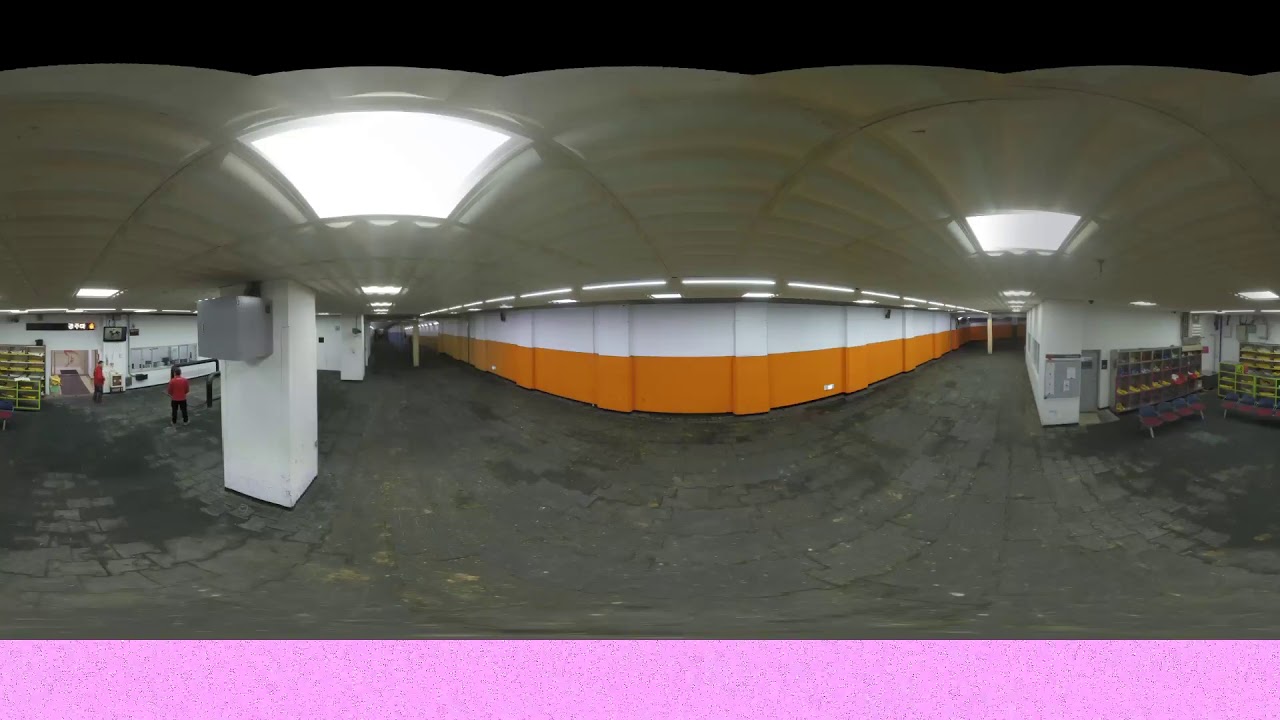The image depicts a spacious industrial or manufacturing plant with a large concrete floor spanning the building. The ceiling is a beige color and features a bubbled roof with large skylights, one closer on the left and one farther away on the right, flooding the interior with natural light. At the foreground on the left, a white pillar stands prominently, topped with a gray electrical or air conditioning box. Just left of this pillar, a small person in black pants and a red t-shirt provides a sense of the building's vast scale. 

Dominating the middle of the image is a semi-circular wall that's white on top and orange on the bottom. This wall curves gracefully from the left, arcs towards the front, and circles back to the right. To the far right, there are another white wall, shelves filled with neon-colored items, possibly shoes, and a couple of benches or seats. Nearby, there is a gray door adjacent to a hallway. The left background of the image features another hallway next to a white wall with several windows. Multiple people can be seen milling about, contributing to the bustling yet organized atmosphere of the space. The image is framed by a pink border at the bottom and a black border at the top.